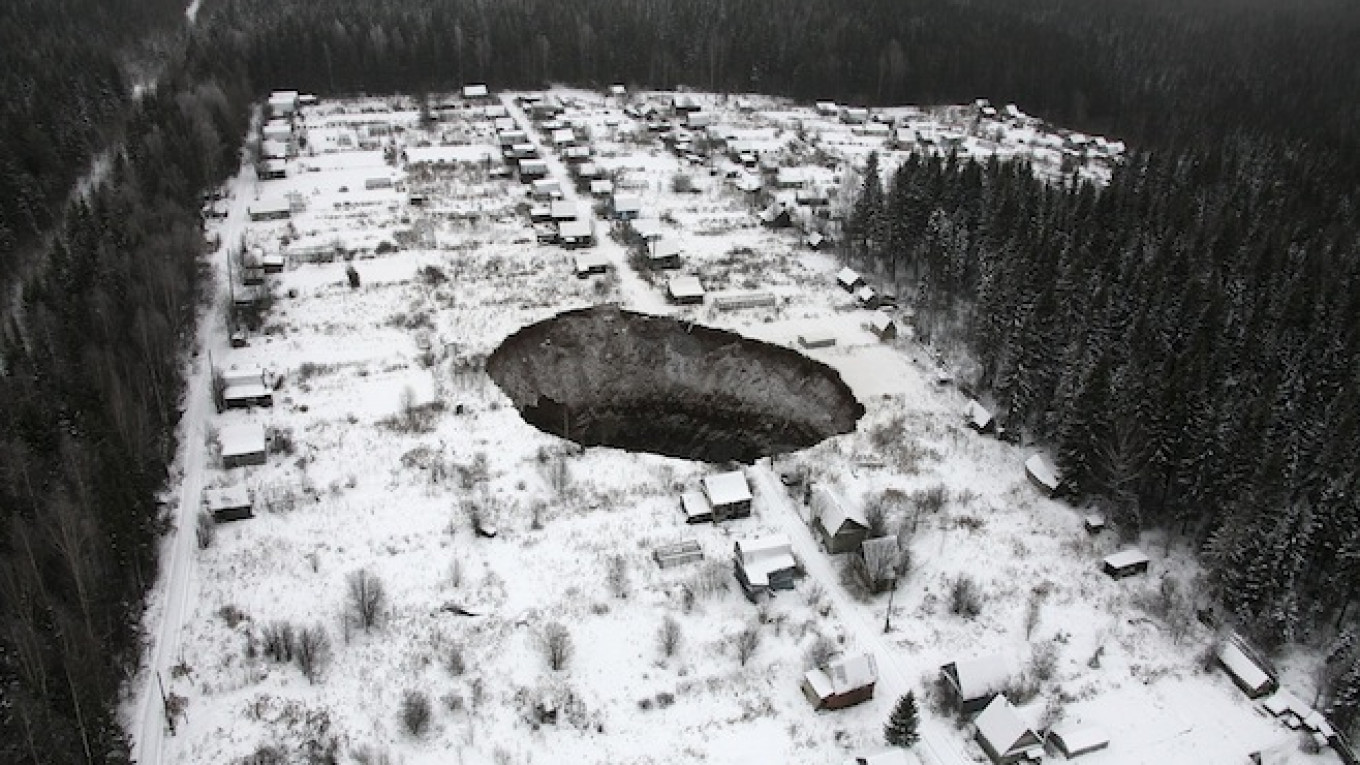This black and white aerial photograph captures a small, snow-covered town nestled within a dense alpine forest, primarily composed of tall pine trees. The scene is somber, almost morose, accentuated by the grayscale palette. At the heart of the town lies a massive, gaping sinkhole, appearing nearly circular and engulfing part of the central roadway. This sinkhole, which seems to be several houses wide, adds an element of distress, suggesting a sudden impact or natural disaster, potentially leading to great loss. The residential buildings, likely cabins, form loose clusters around the central void, with one main road traversing the town from the bottom right to the top left, intersecting the edge of the sinkhole. The tops of the homes and the roads are dusted with snow, adding to the eeriness. Scattered light posts and sparse trees dot the town's layout, while the surrounding dense forest forms an untouched border, enclosing the tragic scene within its natural boundaries.